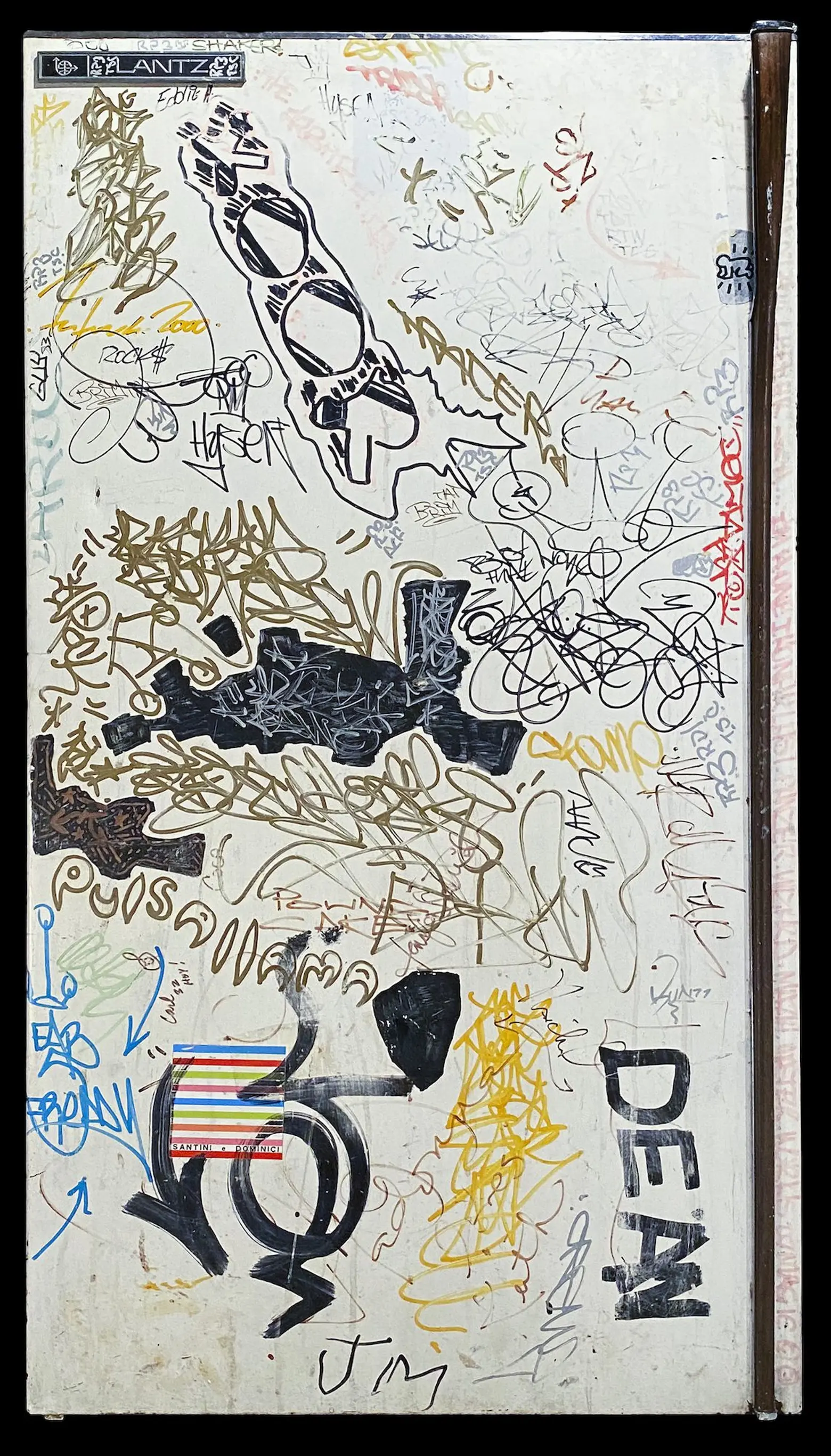The image features a white wooden plank, possibly resembling an old refrigerator with a thin wooden bar running from top to bottom on the right side, which is covered extensively in colorful graffiti scribbles and drawings of various sizes. Predominantly, large bold black marker lines make up much of the visible graffiti, with the name "DEAN" written vertically in the lower right corner and horizontally near the bottom right. The graffiti includes various arrows — a thick black arrow-like squiggle resembling a shield, and other thin arrows pointing left and downward with a multi-colored, striped pattern that seems like a flag. Above these arrows, there are black letters spelling out "P-U-I-S-A-H-A-M-A." The background is mostly white with various colored marker scribbles — including brown, red, yellow, blue, light blue, gold, and purple — creating an eclectic and chaotic mix. Some identifiable shapes include what looks like a rocket ship in the upper left corner. The plank rests against a solid black background, enhancing the vividness and contrast of the graffiti artwork.